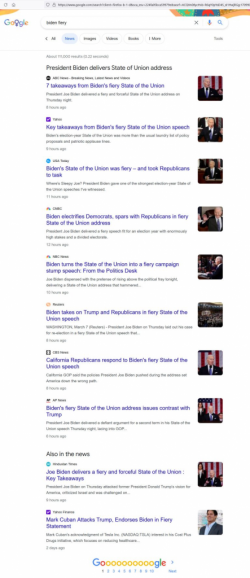A detailed Google Search page is displayed, highlighting the results of a search for "Joe Biden" that prominently feature various images depicting him appearing sleepy. The top of the page showcases the colorful Google logo on the left and another multi-colored icon on the right. The search results include ten different entries, each accompanied by a photo of President Joe Biden looking drowsy. The interface features elements for adjusting visual settings, such as stroke size, with the first option selected and visible in green.